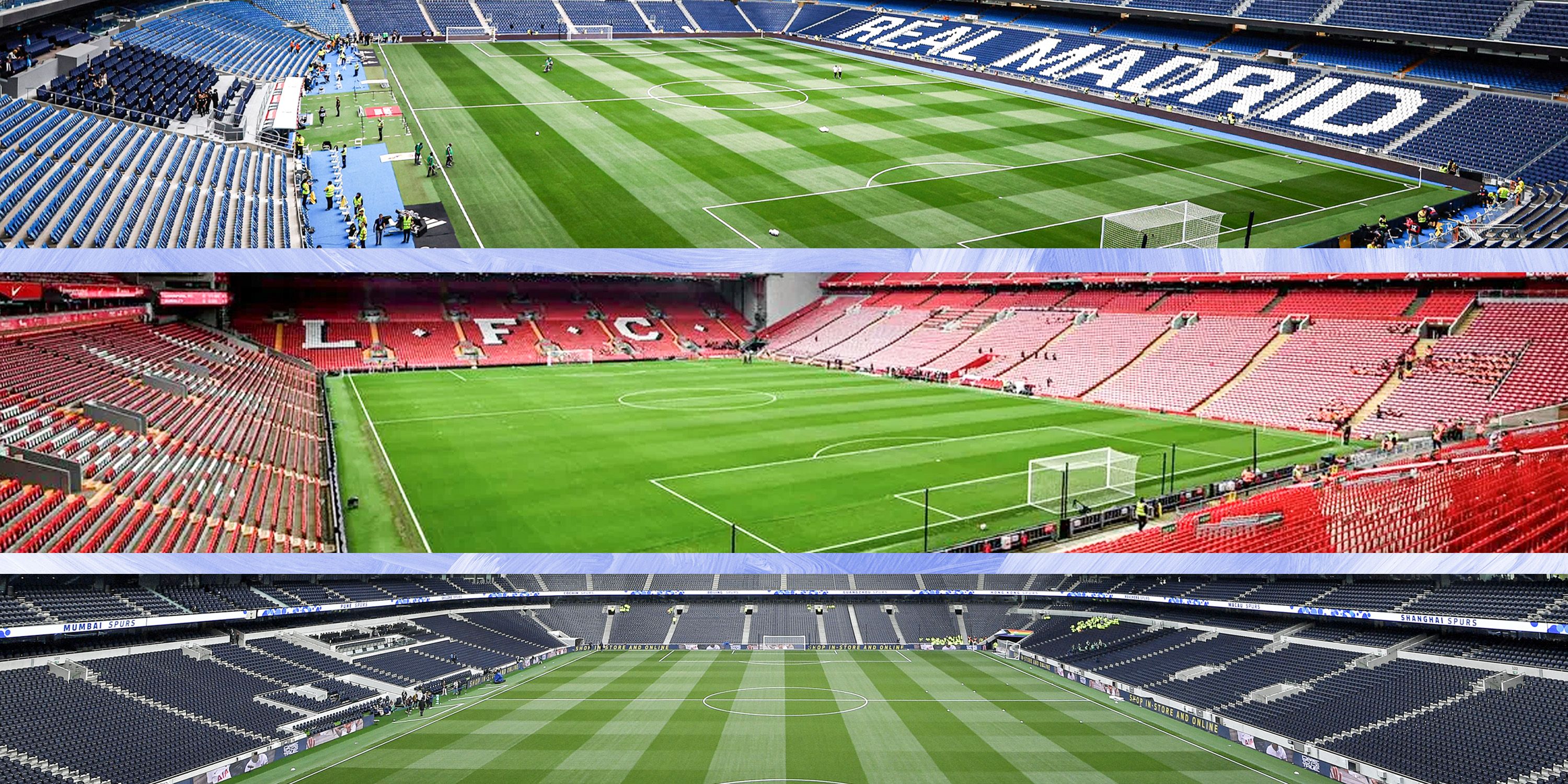The image features three vertically arranged photographs of distinct soccer stadiums. The top photograph showcases a football stadium with lush green grass patterned with vertical and horizontal stripes of dark and light green. The stadium's stands are blue, prominently displaying "Real Madrid" in white letters on one side. The central photograph depicts another football field, also lush with green grass showcasing horizontal stripes creating light and dark green shades. This stadium's stands are bright red with "LFC" written in white letters on one side. The bottom photograph reveals a third stadium with a similarly striped football field of dark and light green grass. The stands here are a dark navy or almost black color, with no text or markings visible. In all photographs, the fields appear empty, though there are a few barely visible people in the lower rows of the bottom stadium.